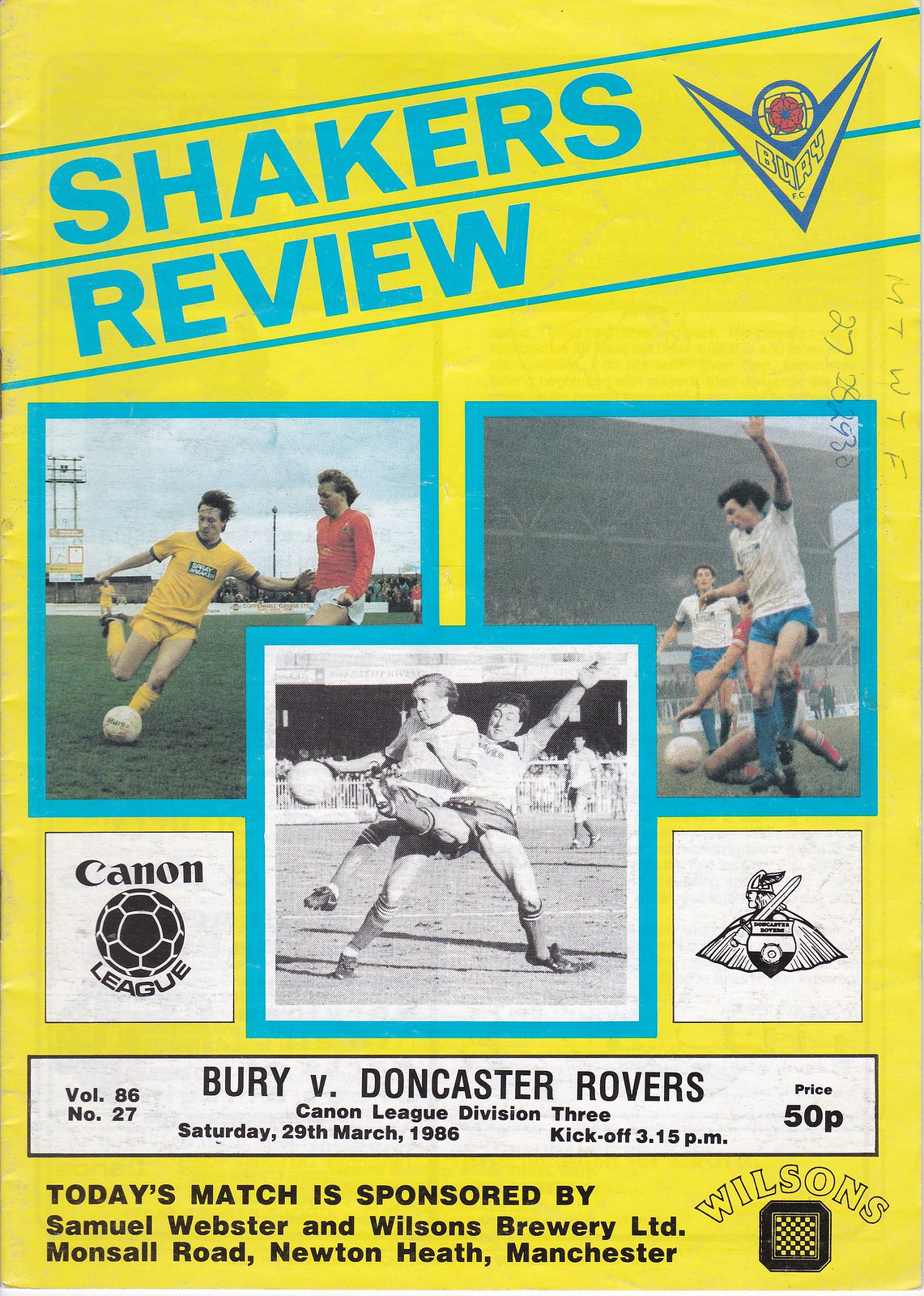The image is of a football magazine titled "Shakers Review," with a predominantly yellow cover and blue text. This edition is Volume 86, Number 27, featuring the match between Bury and Doncaster Rovers in the Canon League Division III on Saturday, March 29, 1986, with a kickoff at 3:15 p.m. and priced at 50 pence. The cover displays three photographs of players mid-action: one showing players in yellow and red, another with players in white shirts and blue shorts, and a black-and-white photo of a goalie blocking a ball. At the top, the title "Shakers Review" is written in light blue, angled upward to the right. There is a distinctive logo at the upper right corner featuring a soccer ball and a "V." To the left of the central bottom image, there's a white rectangle with "Cannon League" and a soccer ball, and to the right, another rectangle depicts a man with a winged helmet and a sword. The bottom inscription in black reads: "Today's match is sponsored by Samuel Webster and Wilson's Brewery Ltd., Monsal Road, Newton Heath, Manchester," with a checkered box and "Wilson's" to the right of the text. Creases are visible on the left side of the magazine, adding to the vintage feel of the program.